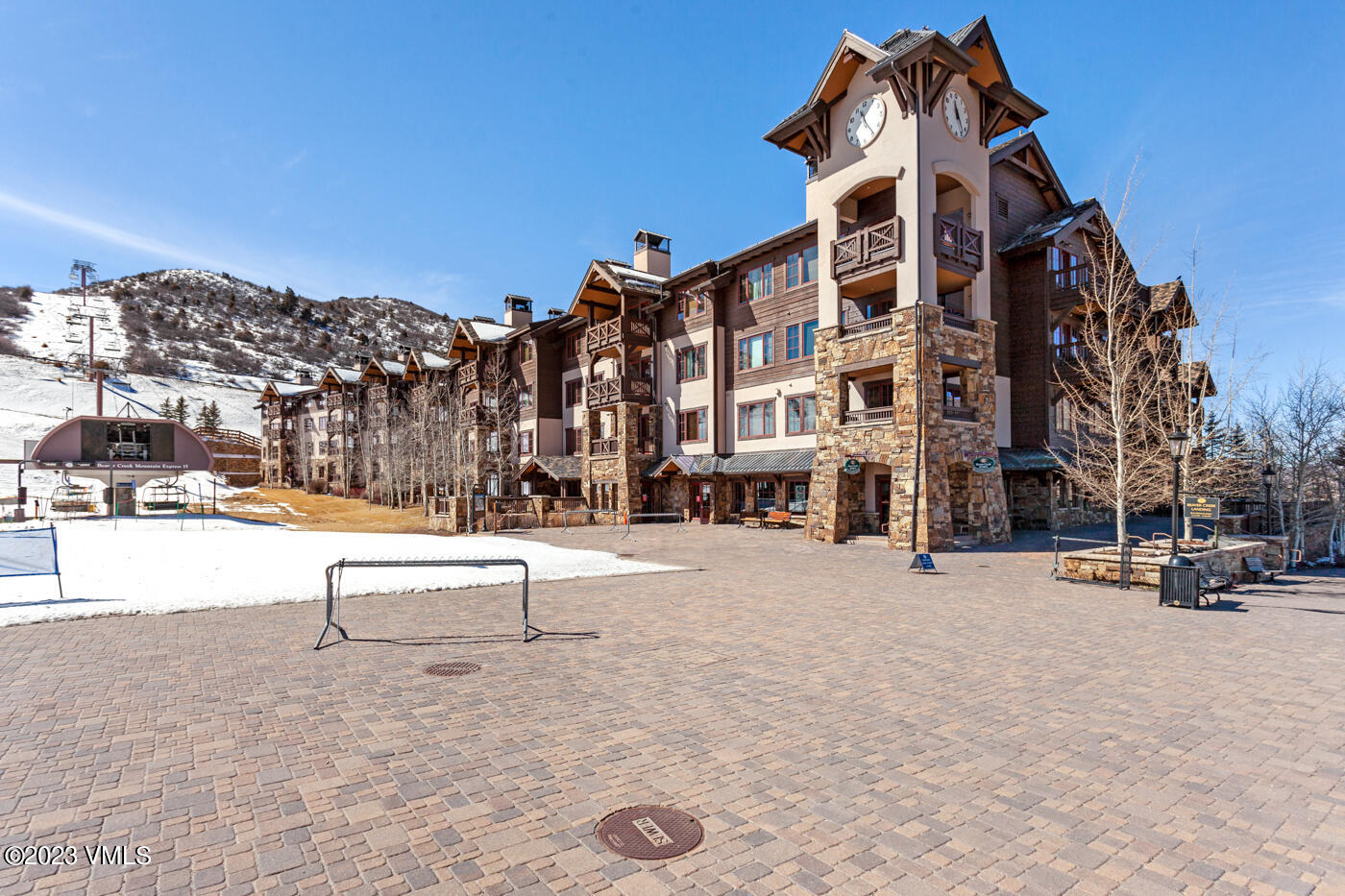The image depicts an expansive outdoor scene at a ski resort nestled at the base of a snowy mountain. The central focus is a three-story hotel or chain of buildings resembling interconnected condo units, with a distinctive clock tower featuring a white clock face with black hands and numbers. This well-maintained structure, possibly historical, showcases a varied color palette of dark to light brown stone veneer, giving the appearance of brick, especially around each tower-shaped entrance. Dark brown wooden panels frame numerous windows and balconies, adding to the rustic charm. 

The plaza in front of the buildings is paved with an assortment of brown and gray stone or brick pavers, extending towards a small cluster of leafless trees, suggesting winter. The landscape transitions towards the rear, where snow-covered ground and patches of brown grass blend seamlessly into the backdrop of the resort. To the left, the scene features a ski lift apparatus with metal support poles and cable cars, indicating this is indeed a ski resort. The hill beyond is dotted with evergreen trees, reinforcing the wintery, alpine atmosphere. Overhead, a partly sunny blue sky with a single white cloud completes this picturesque setting.